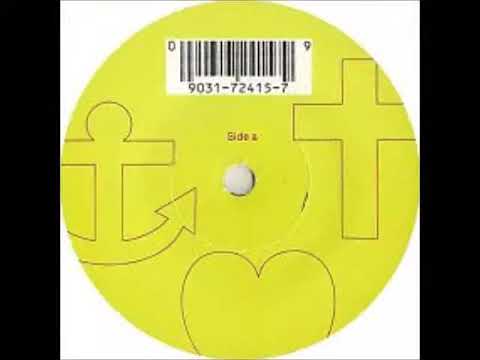The image depicts what seems to be a handmade or vintage album, possibly a record or CD. It features a central yellow circle on a white background, flanked on both sides by black bars. The yellow circle, resembling a CD or record label, includes small, somewhat blurry text that likely reads "side," possibly indicating "Side A" or "Side 2." Above this text is a barcode with the serial number 9031-72415-7. Additionally, the circle contains icons of an anchor, a cross, and a heart. The overall size of the image is approximately 5 inches by 4 inches, and the image quality is of medium resolution. There is no further text to identify the artist or the album.